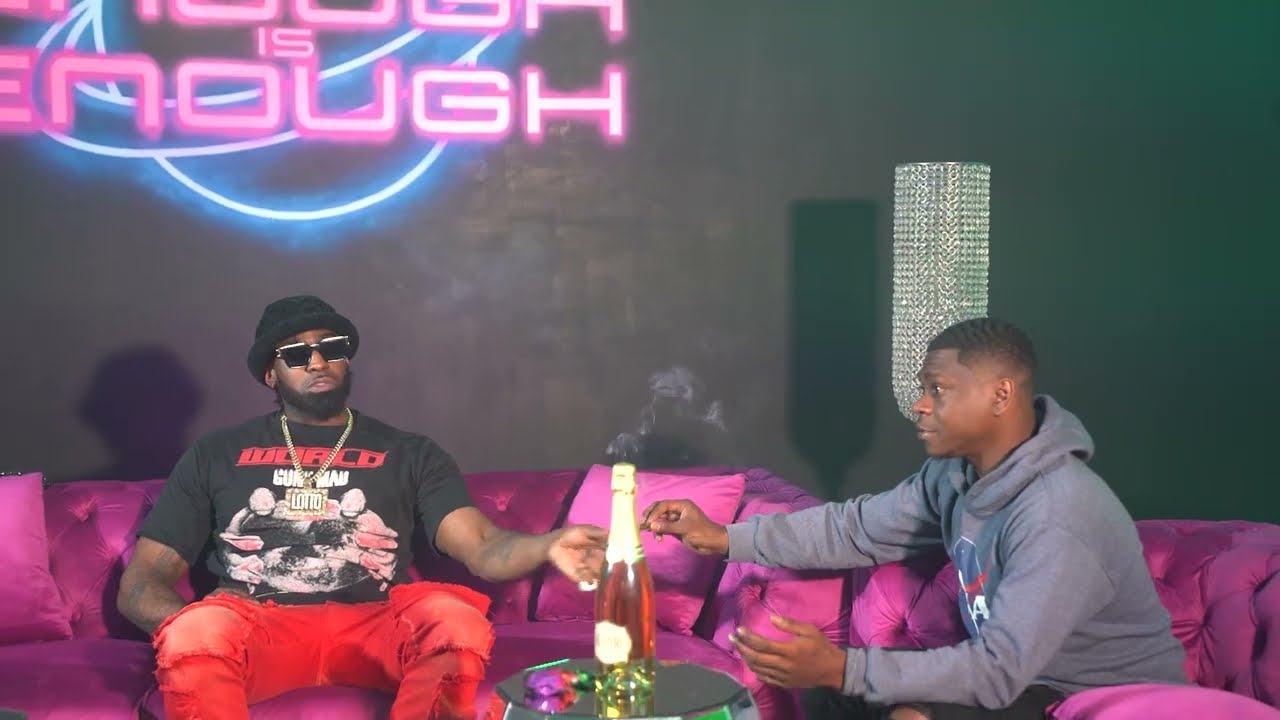In a vibrant indoor setting, two black men are seated on a sumptuous, purplish-pink velvet couch reminiscent of the 80s. The backdrop features a striking black wall adorned with an eye-catching pink neon sign declaring "Enough is Enough," juxtaposed with a vivid LED depiction of Saturn in blue. The air of opulence is heightened by a disco ball-inspired glass table positioned in front of them, which holds an expensive-looking bottle of rose red wine or pink champagne, along with colorful balloons in purple, red, and green hues.

The man on the left, clean-shaven with a short fade haircut, sports a grey NASA hoodie prominently displaying the NASA icon, paired with distressed, bright red pants that have a layered design. He accessorizes with a gold chain, thick black sunglasses, and a black bowler-type beanie. The man on the right, wearing a black shirt with unreadable red and white lettering, also dons sunglasses and a black beanie. He extends his right hand to pass a lit blunt to the man on the left, who receives it with his left hand amidst the swirling gray smoke.

Adding a touch of elegance, a crystal chandelier-like lamp glimmers subtly behind the man on the right. The overall ambiance suggests a fashionable, possibly interview-like scenario, evoking the aura of an intimate, stylish gathering or a candid moment shared between friends.